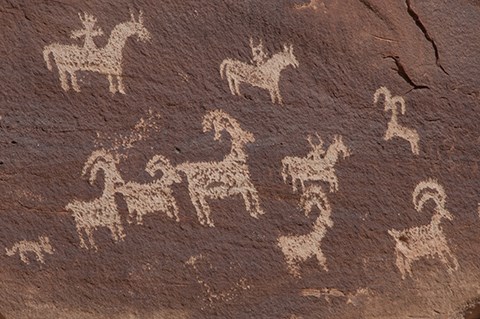The image depicts a small, horizontally oriented rectangle, showcasing what appears to be ancient Stone Age cave drawings on a dark, dirty stone surface. The scene is intricately detailed with numerous carved animals and human figures. On the top left, there is a llama with a rider, followed by three goats beneath it. To the right of these, at the top, is a person riding a horse, with another horse and rider directly below. Beneath the second horse, a goat with long horns is carved. All animals appear to face right, except a goat at the top right corner, which faces left. 

Throughout the carving, various animals with antlers are present, including larger and smaller ones. Notably, in the bottom right corner, there is an animal with a large tail, and in the bottom left corner, behind the antlered animals, a small creature is visible. The detailed carvings convey a scene rich with movement and interaction, providing a fascinating glimpse into the artistic expression of early humans.